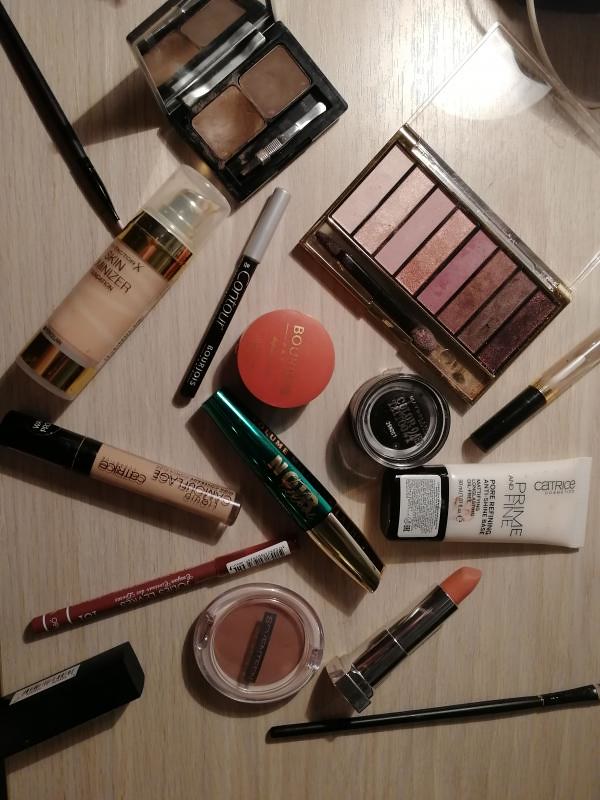The top-down photograph showcases an array of makeup and beauty products meticulously arranged on an off-white, wood-grain surface. In the top-right corner, an unidentified object casts a shadow, adding a hint of mystery. 

In the top-left portion of the image, an open makeup case reveals two distinct shades of brown, accompanied by a mirror embedded in the lid. Just below, a palette featuring eight colors transitions seamlessly from a delicate light pink to a deep, dark brown.

Moving downward, we encounter a container of skin sanitizer. Directly beneath this, there appears to be a lipstick. At the bottom center, a round container holds another type of makeup. 

Above this, several eyeliner pens are neatly placed, ready for precision application. Slightly higher, two round containers, likely lip gloss, add a touch of shimmer to the collection. 

To the right, a tube labeled "Prime and Fine" in black on a white background makes a statement. Finally, completing the bottom of the frame, another elongated pencil-like item is poised for use, an essential tool for makeup application.